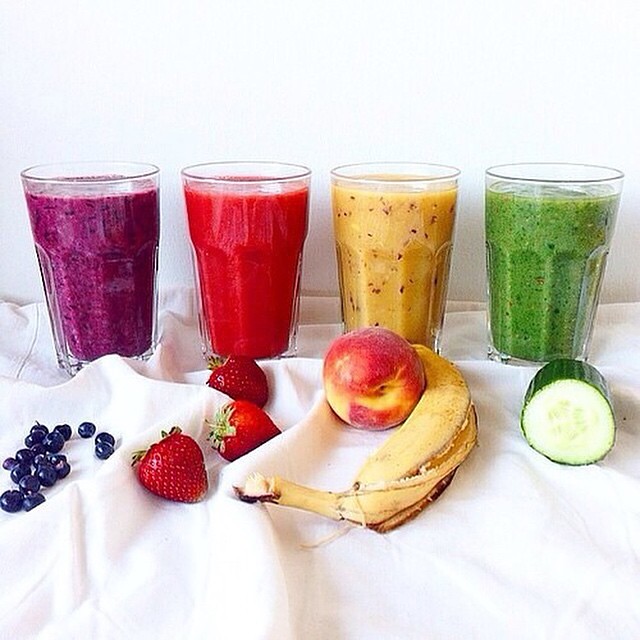This image features four clear glasses filled with vibrant, freshly made fruit and vegetable smoothies, meticulously arranged from left to right on a smooth, white cloth backdrop with a plain white wall behind them. The first glass holds a rich purple smoothie, accompanied by whole blueberries scattered in front, indicating its blueberry composition. The second glass contains a vivid red smoothie, with fresh strawberries displayed prominently in front, signifying a strawberry smoothie. The third glass houses a bright yellow smoothie, placed behind a peach and a peeled banana, illustrating a peach-banana blend. The final glass on the right presents a green smoothie, with a sliced cucumber in front, representing a cucumber smoothie. The fruits and vegetables are thoughtfully arranged to visually represent the ingredients of each smoothie, suggesting a high-quality, possibly commercial presentation.